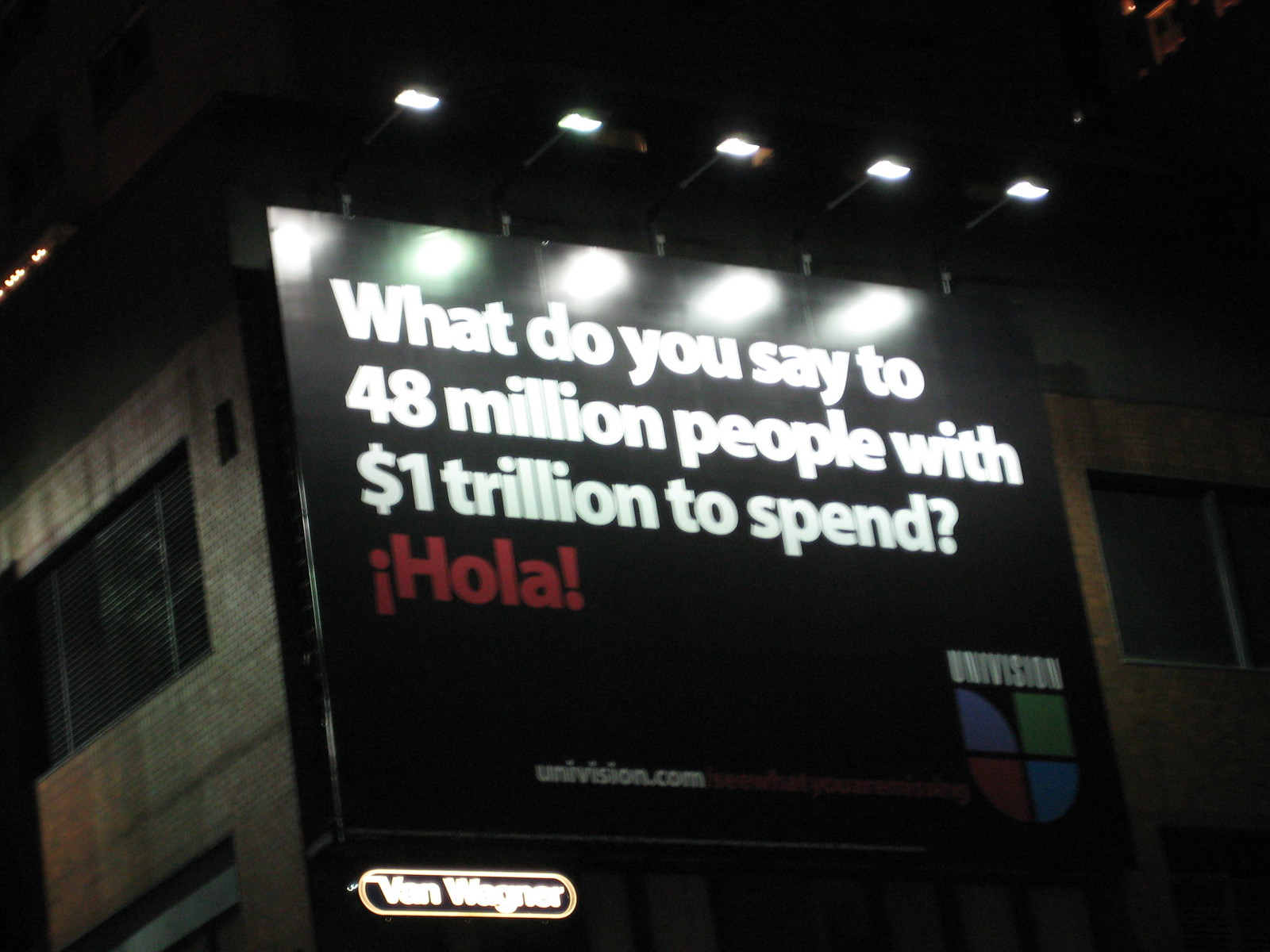The image features an advertisement billboard prominently displayed on the side of a gray, stone-like building. It's nighttime, and the scene is shrouded in darkness, illuminated primarily by five lights positioned above the billboard, casting their glow downward. The billboard's background is entirely black, providing a stark contrast to the text and logos.

The message on the billboard reads: "What do you say to 48 million people with $1 trillion to spend?" This text is rendered in crisp, white lettering and occupies the top half of the billboard. Below this, in the fourth row, is the word "Hola" in bright red letters, framed by an upside-down exclamation mark on the left and a right-side-up exclamation mark on the right, emphasizing the greeting.

In the lower corner, the logo and name of Univision, a Spanish-language television network, are displayed. The Univision logo is multi-colored, featuring segments in blue, purple, green, and red. Below the logo, the website "univision.com" is written in white lettering.

At the bottom of the billboard, the name "Van Wagner," presumably the billboard's creator, is printed in white lettering within an oval shape, signifying the designer's signature touch.

This detailed and strategically illuminated billboard aims to capture attention and deliver a powerful message to the viewers, leveraging the visibility offered by the unique placement on the building’s side.